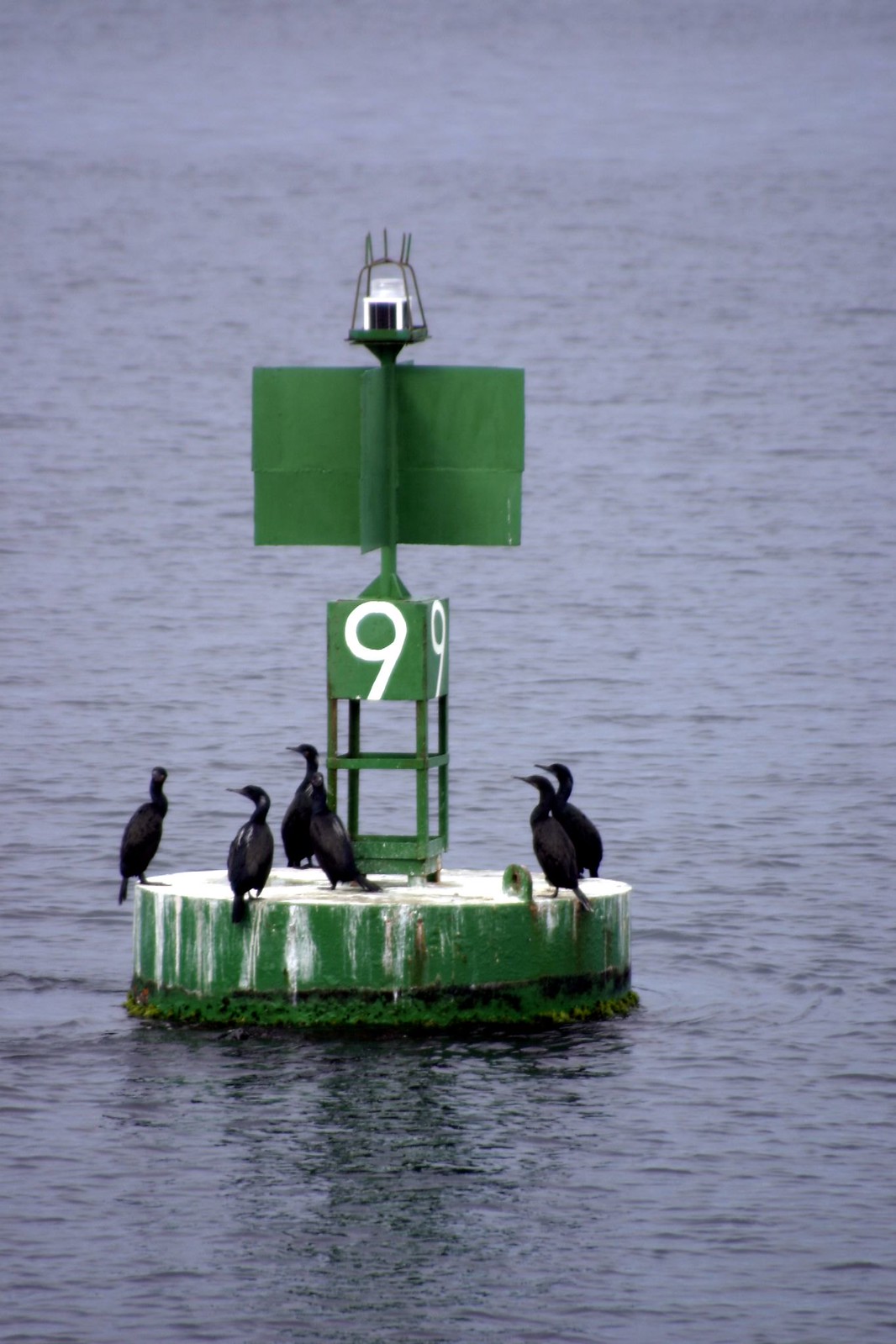The image captures a green buoy floating in a calm, grayish-colored body of water. The buoy is prominently marked with the number nine on multiple sides and appears to have a light on top. It also features a sign in green, though the text is not visible from the angle the photo was taken. Perched on the buoy are several large black birds—four to the left and two to the right of the number nine—all facing the same direction as if anticipating something. The buoy is streaked with white, likely bird droppings, indicating the birds' regular landing practice. The scene is set in an isolated location, surrounded by water with no land in sight, and captured within a rectangular frame, emphasizing the tranquility of the setting with barely any waves, just gentle ripples on the water's surface.